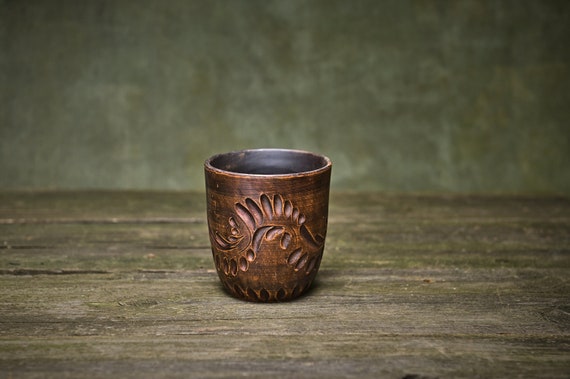In this detailed photograph, a small, intricately designed brown cup is prominently featured. The cup, which appears to be crafted from wood, showcases a beautifully carved pattern of leafy shapes, circles, and ovals that wave elegantly along its surface. The exterior is a consistent brown, while the interior has a contrasting darker brown or black hue. The cup is placed on a visually aged, gray wooden tabletop, consisting of several distinct boards, and is illuminated by overhead light, bringing its detailed carvings into sharp focus. The blurred background features a smudgy, olive-green wall, adding depth and contrast to the overall composition. The photograph is sharply focused on the cup, highlighting its meticulous craftsmanship and textured surface.